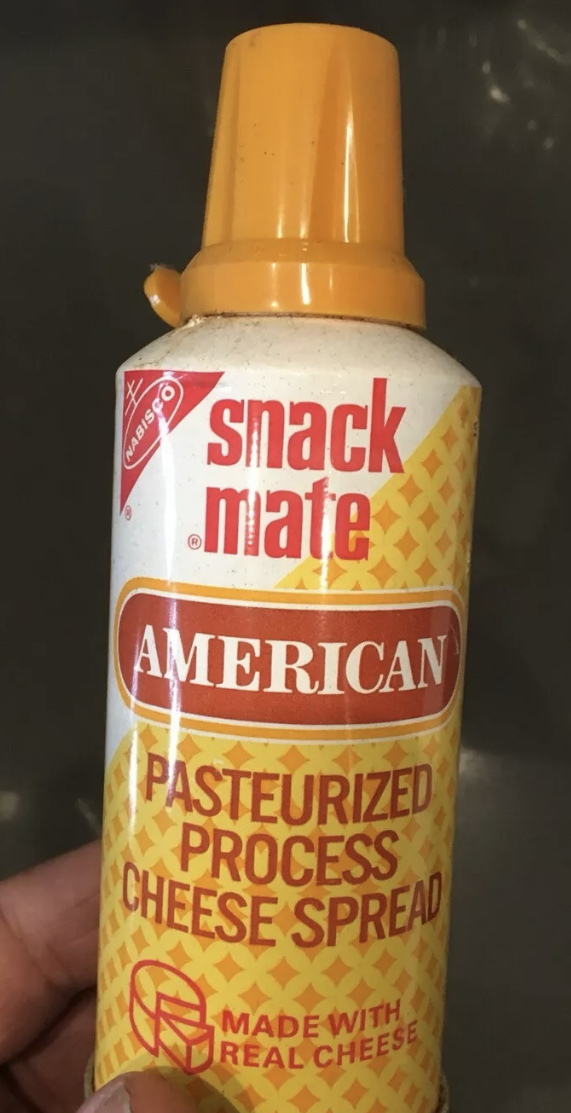A close-up image of a snack food reveals a well-worn can of cheese being held by a man's fingers in the bottom left corner. The top of the can, capped with a light orange lid, is dusted, indicating it has likely been sitting in a pantry, untouched, for some time. The upper half of the can features a white background, while the lower half showcases a vibrant yellow background with orange diamonds. Prominently displayed in red lettering at the top is the brand name "Snack Mate." In the top left corner, the Nabisco logo is visible, also in white lettering on a red background. Centrally placed in red on a white background is the word "American." Below this, additional text reads, "Pasteurized Processed Cheese Spread Made with Real Cheese," providing further details about the product.